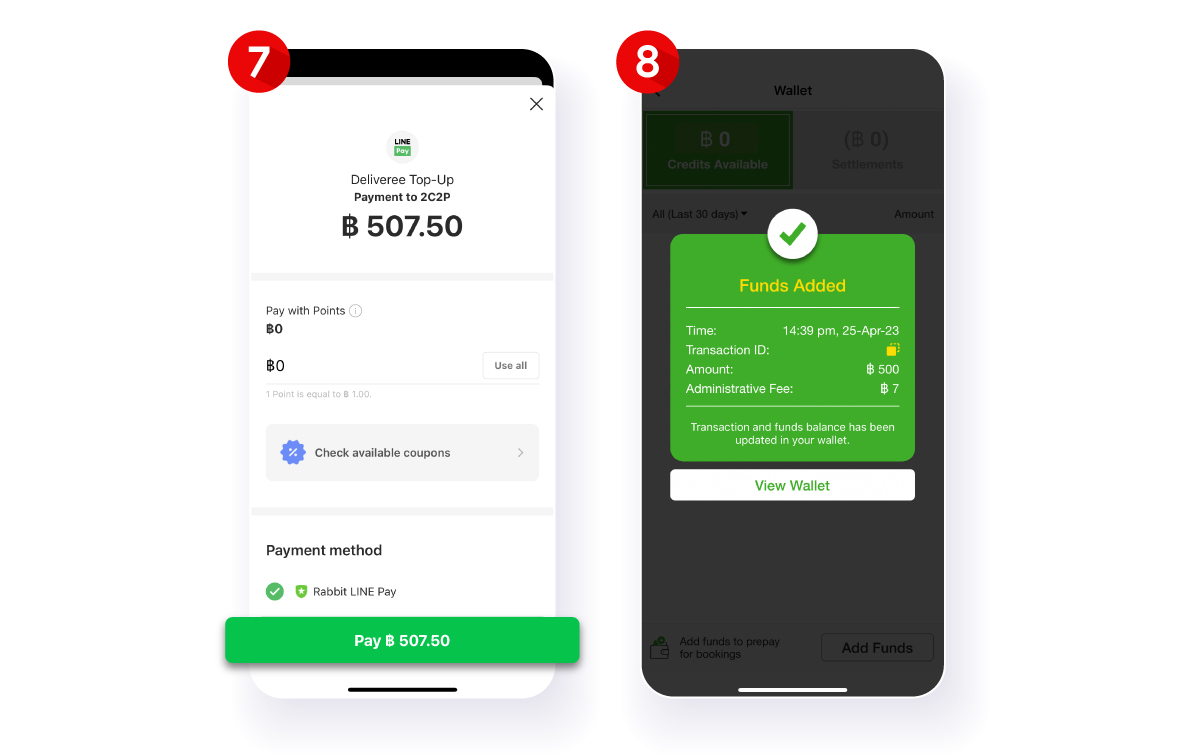This image is a detailed screenshot of a mobile payment process interface, displayed across two phones side-by-side on the left side of the screen. In the top right corner, there is a red circle with a white number 7 inside it. A black border runs horizontally across, with a thin gray border outlining the top, left, and right sides of the interface, while the center has a white background.

At the top right corner within the main interface, a black 'X' icon is visible. Moving down to the center left, there is a gray circle with the word "Line" in bolded black font at the top, accompanied by a green tab below it that reads "Pay" in white. Beneath that, black text reads "Delivery Top-Up" followed by "Payment to 2C2P" with the amount "507.50" displayed below.

A thin gray border separates the amount from the next section, which reads "Pay with Points" on the left side. Adjacent to this text is a small gray circle with a gray 'i' icon inside it. Below this, bolded text shows "0" followed by "0". On the right side, there is a white tab with the text "Use All" in gray. A large gray tab spans the width of the section, featuring a blue circle with a white percentage sign next to the black text "Check Available Coupons". Another thin gray border follows this section.

In the next section down, positioned on the left side in bolded black text, is the label "Payment Method". This section includes a green circle with a white checkmark, and a green shield icon with a white star. Beside these icons, black text reads "Revit Line Play". Below this section, a large green button stretches across the interface, with "Pay 507.50" displayed in white at its center.

To the right side of the interface, the background has a grayish tint due to a pop-up tab. In the top left corner of this pop-up, a big red circle with a white number 8 is visible. The black text reads "Wallet". The pop-up tab itself is green, featuring a green checkmark icon at the top. Below this, in yellow text, it states "Funds Added", followed by detailed information beneath. At the bottom, there is a white search tab labeled "View Wallet" in green.